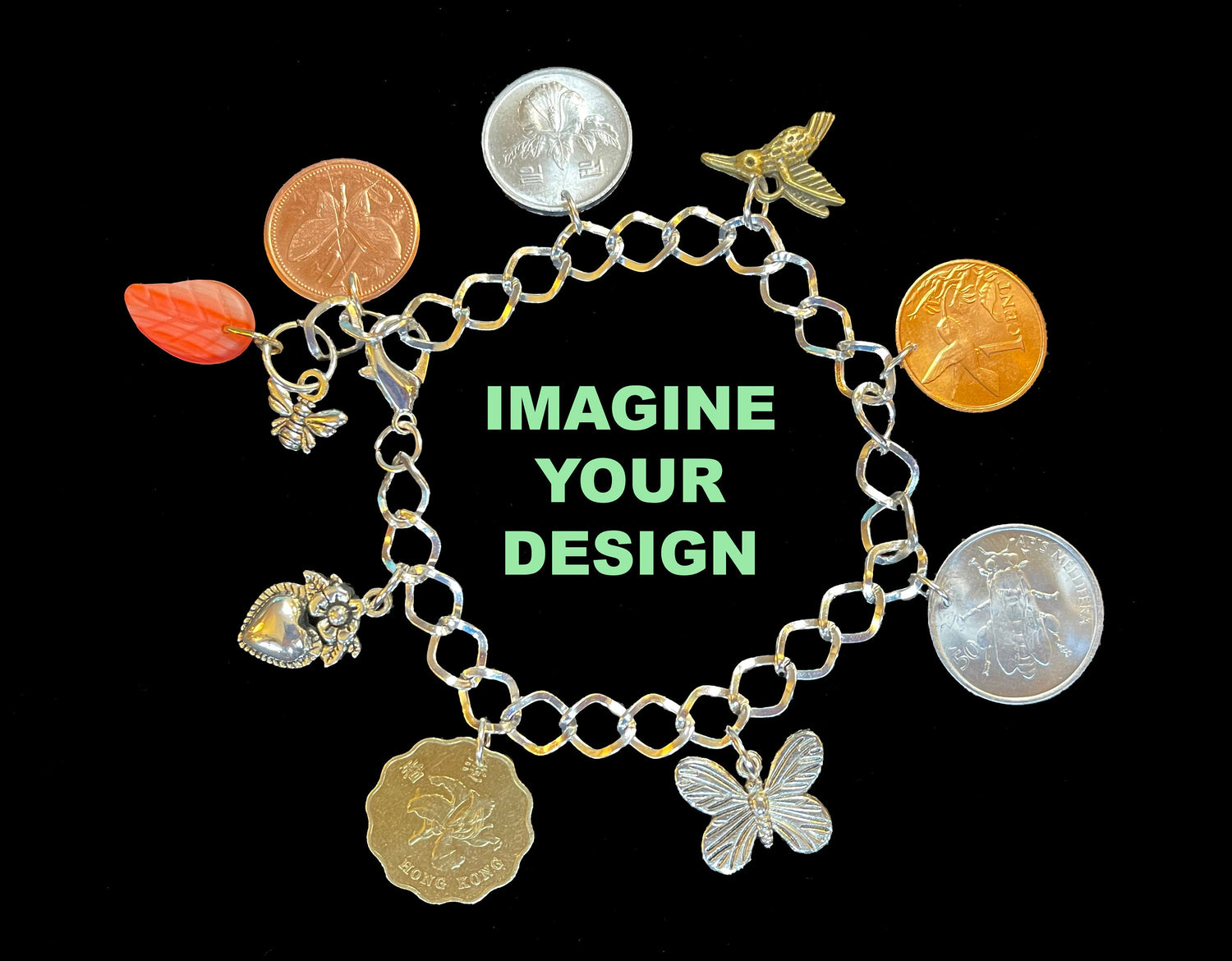The image depicts a charm bracelet laid flat against a plain black background. Encircling the light green text in the center that reads "IMAGINE YOUR DESIGN" in capital letters, the bracelet features several meticulously detailed charms. The bracelet itself is composed of silver O-shaped links. Starting from the clasp on the left, the first charm is a silver bee and a red leaf sharing the same ring. Next is a copper-colored coin adorned with the image of a butterfly. Following that is a silver coin, which appears to exhibit Korean or Chinese writing and features an iris or hibiscus flower. The next charm is a brass-colored hummingbird, succeeded by another copper coin that also portrays a hummingbird and is labeled "one cent." Adjacent to that is a coin featuring a fly and marked with the number "50," the specific currency is indistinguishable. Continuing around the bracelet, there is a small, silver-colored butterfly charm. Next is a gold-colored, scallop-edged coin with "Hong Kong" inscribed on it and a flower in the center. The last charm is a heart with a flower and leaves positioned above it, hanging delicately. This rich array of charms, ranging from intricate coin designs to detailed depictions of animals and flowers, beautifully embellishes the bracelet.